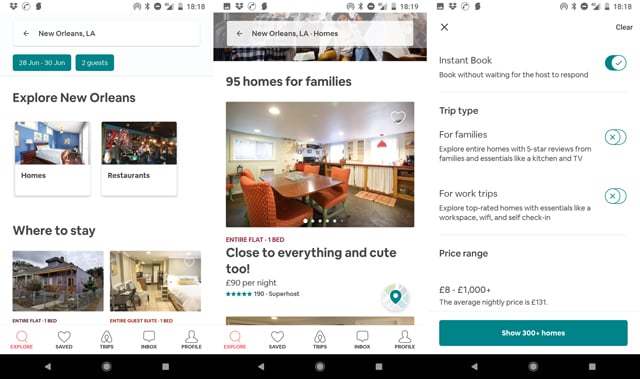A composite image composed of three merged phone screenshots, all featuring bright white backgrounds, showcases a hotel booking app. The screenshots, aligned side by side, give a misleading initial impression of being a single large picture. The repetitive navigation bar at the bottom of each screenshot reveals the true nature of the composite. 

The app displayed in the screenshots appears to be used for booking accommodations in New Orleans, Louisiana. The search parameters set include a stay from June 28th to June 30th for two guests. The middle screenshot highlights a selected listing: an "Entire flat, one bed, close to everything and cute too" priced at £90 per night. This detail suggests the app is either a UK-based service or the user is located in the UK, resulting in the price being displayed in British Pounds.